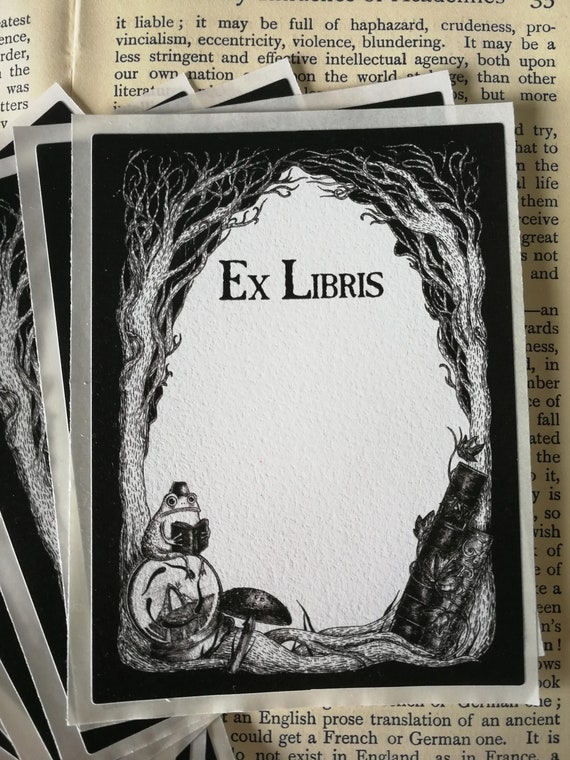In the image, a detailed Ex Libris card is positioned on top of three other identical cards, all of which rest on an open book. The Ex Libris card, featuring a black and white design, depicts a frog comfortably perched on a crystal ball, engrossed in reading a book. Surrounding the frog are detailed, leafless trees that frame the scene like a mystical forest, with a mushroom nestled at the base of the crystal ball. The card prominently displays the words "Ex Libris" in bold black letters at the top. The background is black, giving the scene a dramatic contrast. In the intricate environment, branches and cylindrical structures entwined with flowers add to the surreal atmosphere. The underlying book, appearing to be old with partial sentences visible, mentions phrases like "liable" and exhibits page numbers that could be 55 or 33. The combination of the cards and the book creates an intriguing blend of mysticism and literary charm.